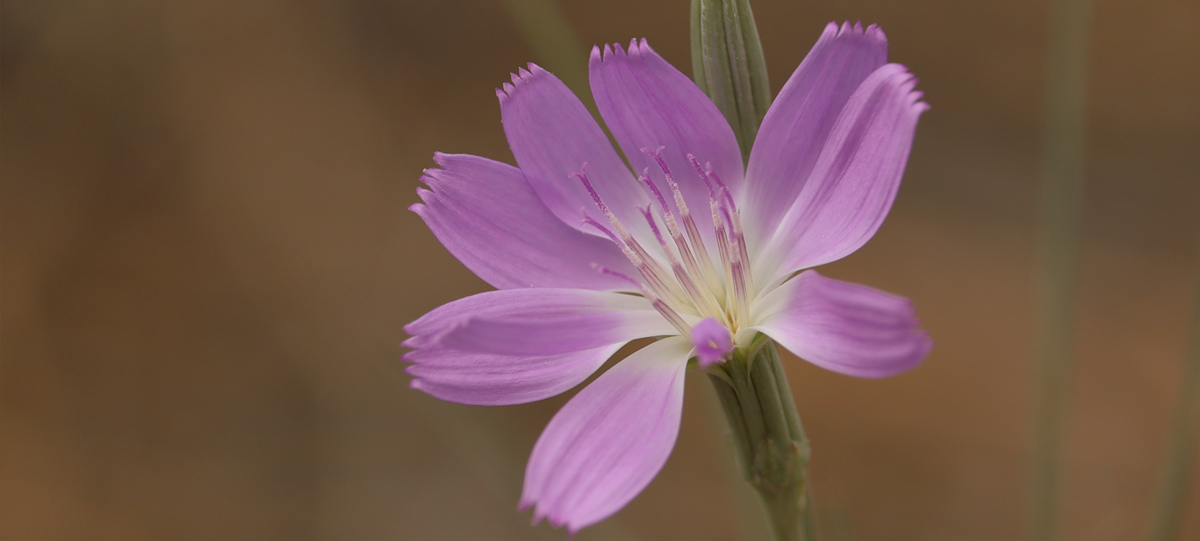This close-up photograph captures an intricate zoomed-in view of nature. On both the left and right sides, the image becomes slightly blurred, with the right side showing a brownish hue. Amidst the blur, green stems are visible, suggesting a connection to other, less discernible flowers. Dominating the image is a flower, whose stem is barely visible due to the extreme close-up. The focus is on the flower’s interior and its petals. The petals are predominantly purple, transitioning to white towards the center. Delicate, sprout-like lines emanate from the middle, forming a pattern that alternates between white and purple. The tips of these sprouts are a darker purple, contrasting subtly with the lighter petal hues.